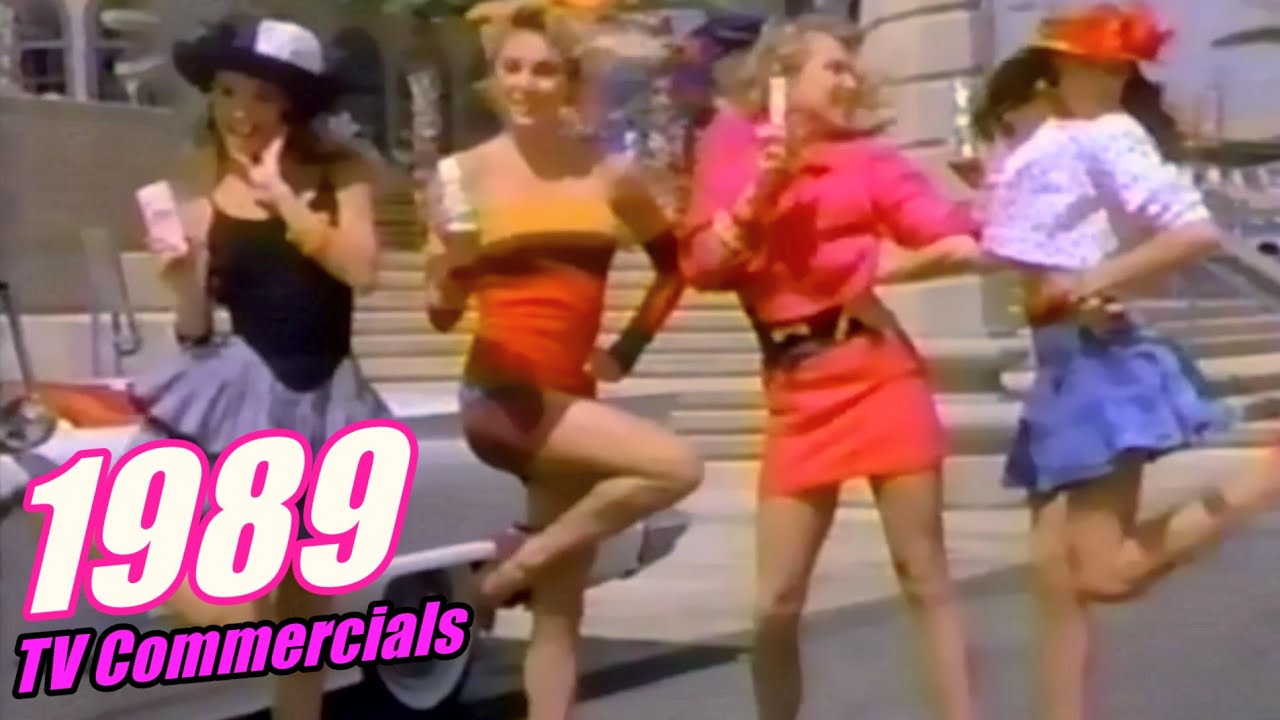The screenshot from a 1989 TV commercial, as indicated by the white text with a pink outline and purple text with a black outline in the bottom left corner, features four Caucasian women posing in colorful outfits. The woman on the far left wears a black tank top, a light blue skirt, and a black-and-white hat. The second woman is dressed in a strapless dress with red and brown stripes. The third woman sports a pink outfit that includes a long-sleeve top and a mini skirt, accessorized with a black belt. The woman on the far right dons a white polka-dot top with sleeves rolled above the elbows, a blue jean skirt, and a red hat. All four women are standing in front of a white vintage car, with a staircase and a large stone building in the background. The old and slightly blurry image captures them in dynamic poses reminiscent of 80s TV commercials.